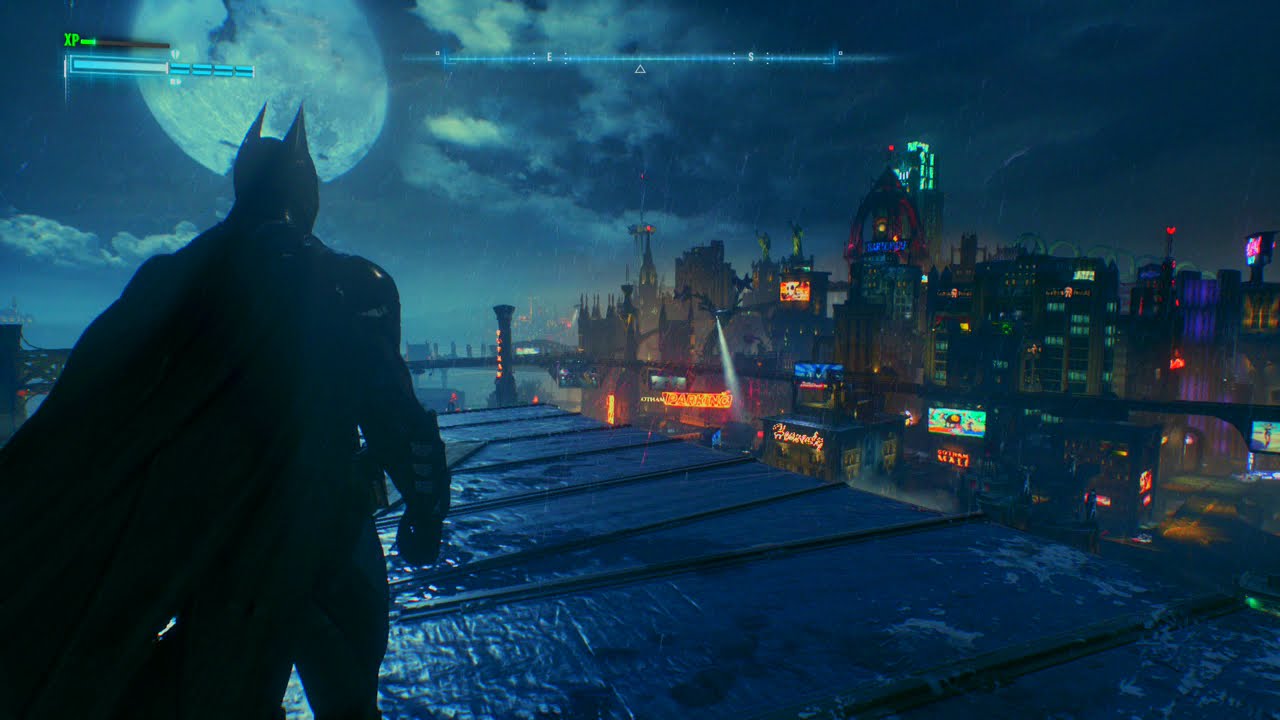A screenshot from a Batman video game captures a dramatic nighttime cityscape. Batman, clad in his classic black suit with the iconic two-pointed cowl and cape, stands on a metallic rooftop to the left of the image. Facing away from us, he assumes a poised, ready stance with his arms by his sides. The rooftop appears wet, suggesting rain, with metal sheets running horizontally across its surface. Overhead, a large full moon, partially obscured by clouds, bathes the scene in a haunting glow, accentuated by the reflection off the wet roof.

Above Batman and to the left, a light blue health bar and a green XP bar are visible on the game interface. To the top right of Batman, a compass display indicates his orientation. In the distance, a bridge leads towards the vibrant and dense Gotham City skyline. The cityscape features predominantly dark skyscrapers, some adorned with glowing orange signs, green-lit windows, and a scattering of other neon hues like pinks and greens. The illuminated buildings contrast with the dark skyline, creating a colorful and atmospheric depiction of Gotham at night.